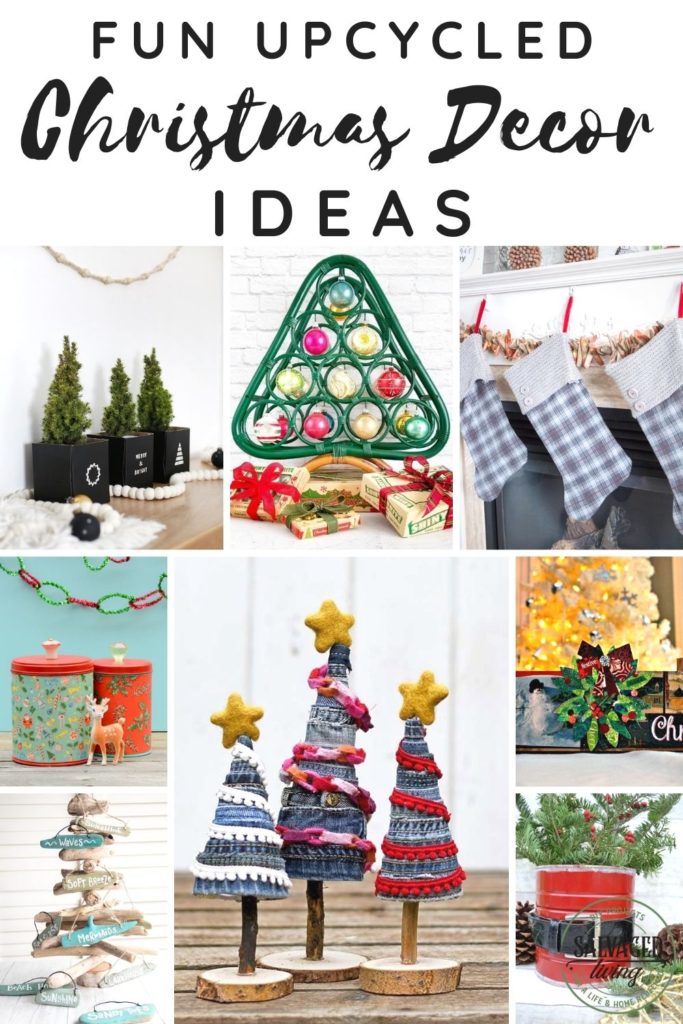This composite photograph, titled "Fun Upcycled Christmas Decor Ideas," features eight individual images showcasing creative and colorful DIY Christmas decorations made from recycled materials. The top left image displays numerous miniature Christmas trees set upon black boxes, adorned with white beads that mimic snowfall. To the right, a photograph highlights a green plastic frame elegantly draped with dangling ornaments. An image of charming homemade Christmas stockings hangs from a festive mantle, capturing the warmth of holiday traditions. There are canisters wrapped in festive Christmas paper, reflecting a clever reuse of everyday items. Another photo depicts small Christmas trees creatively crafted from scraps of denim and felt, emphasizing sustainable holiday decorating. Additionally, a striking tin can painted red and fashioned with a belt transforms it into a Santa Claus decor piece, beautifully illustrating the theme of upcycling. Overall, the collage presents an array of inventive and sustainable ideas for Christmas decor, making delightful use of recycled materials.